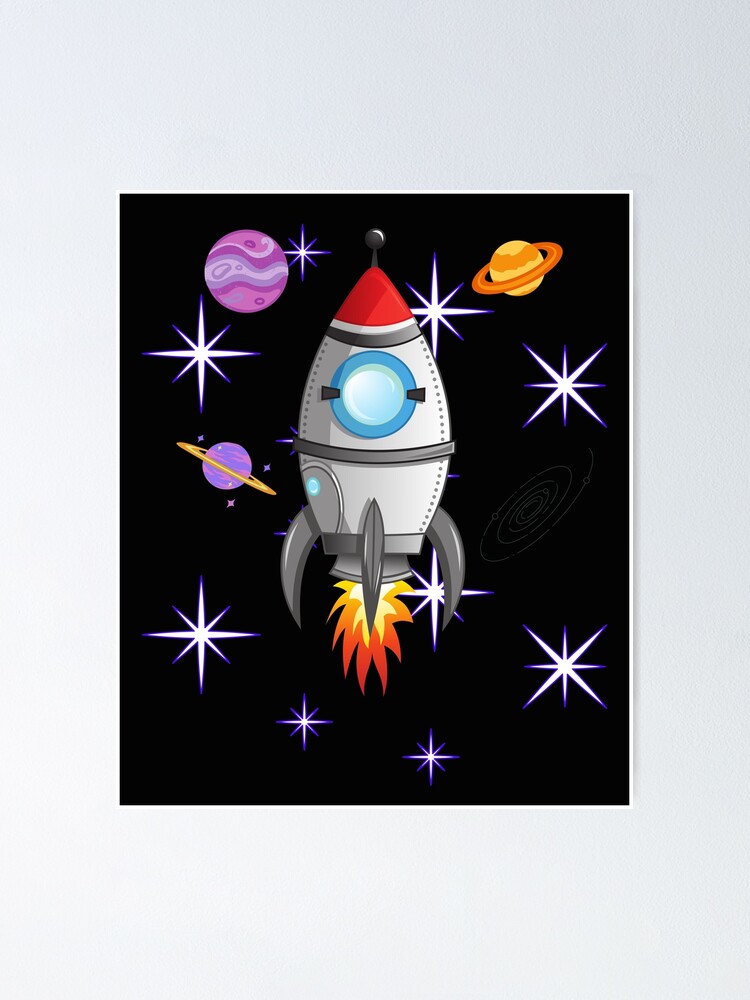The image features a computer-generated artwork of a vertically aligned, rectangular picture set against a solid light gray background. At the center is a black square filled with tiny white specks, representing a starry space. The primary focus is a cylindrical rocket with a red tip that includes a protruding circular knob. The rocket's body is predominantly white with gray stripes and two silver rings, one near the top and one midway down. It also has a bulge along its sides that tapers into a trio of slightly curved, pointy silver legs at the bottom. A blue circular window, secured by two black pins, adorns the middle of the rocket.

Emitting from the bottom of the rocket are vibrant yellow and orange flames, signifying thrust as the rocket ascends. Surrounding this ascending rocket are several celestial elements: a yellow planet with an orange ring in the top right, a purple planet adorned with varying shades of purple swirls in the top left, and another purple planet with a yellow ring in the left middle. The black space backdrop is dotted with larger white stars shaped like asterisks with blue tips, creating a lit-up appearance. The artwork as a whole depicts a dynamic scene of space exploration, with the rocket powering through a cosmic landscape.